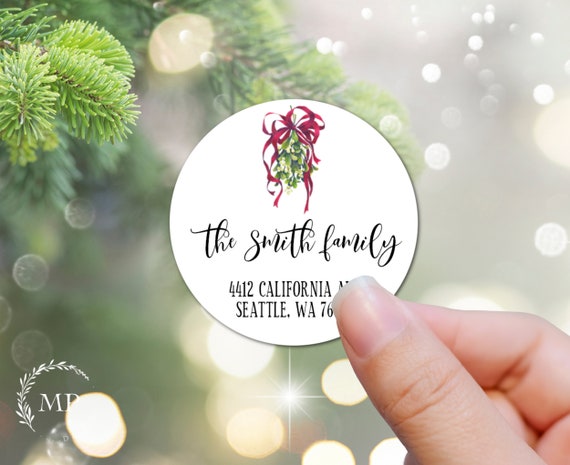This is a high-resolution close-up photograph of a festive Christmas ornament being held by a pale hand, indicating the hand belongs to a white or Caucasian individual. The ornament is white and circular, adorned at the top with a rich maroon/red ribbon tied in multiple bows, from which green foliage, likely mistletoe, hangs. The ornament has black lettering that reads "The Smith Family" in a stylized script, with the address "4412 California Avenue, Seattle, Washington" underneath. However, the zip code is obscured by the thumb of the hand holding the ornament, which is pinching it between the thumb and pointer finger. In the background, there are out-of-focus bright lights and hints of pine tree branches, contributing to the holiday ambiance. Noticeably, in the lower left corner of the image, there is a white spray design featuring the capital letters "MP" possibly encircled by a white illustration resembling a wreath, adding another layer of holiday decoration.